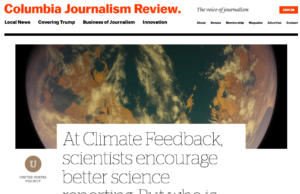The image depicts the homepage of a website titled "Columbia Journalism Review." At the top of the page, a black navigation bar hosts several tabs, including "Local News," "Covering Trump," "Business of Journalism," and "Innovations," among others. The main feature of the page is an article headline that reads "At Climate Feedback, Scientists Encourage Better Science," on a white background with black text. The accompanying image is a view of Earth with vibrant blue oceans, brown land masses, and white clouds. The logo "Columbia Journalism Review" is prominently displayed in orange font on the black bar, along with an additional orange button. Below the navigation bar, there is some cursive writing in black text, further adding to the rich detail and navigational ease of the homepage. The overall background of the webpage is predominantly white, with various sections accessible for users to explore.